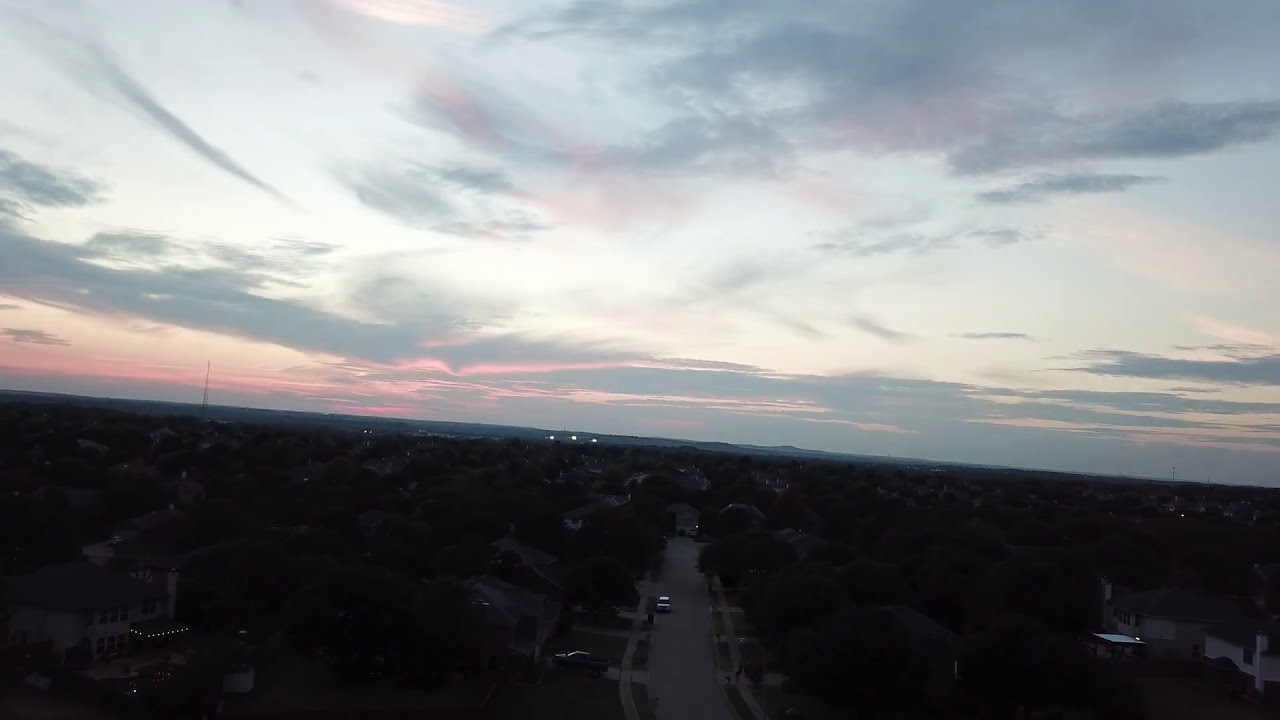This aerial image, taken at dusk, reveals a serene residential area under a captivating sky that occupies around 60% of the frame. The sky, an enchanting blend of light blue, dark blue clouds, and pink hues, suggests the approaching nightfall. The image is slightly tilted to the right, adding a dynamic angle to the scene. Beneath the colorful sky, the ground area appears dim, casting the town or city in shadow. 

In the foreground, a white road stretches toward the back of the image into what seems to be a cul-de-sac. Along the road, houses and trees line both sides, some with lighted roofs or porches, enhancing the evening's tranquility. The left side prominently features a house with lights on the edge of its roof, parked in front is a white car, providing a clear focal point. Other vehicles are sparingly visible on the road, hinting at a quiet, settled community. Toward the far end, in the right-hand side of the background, a hint of a hill or mountainous range is discernible, adding depth to the twilight scene.